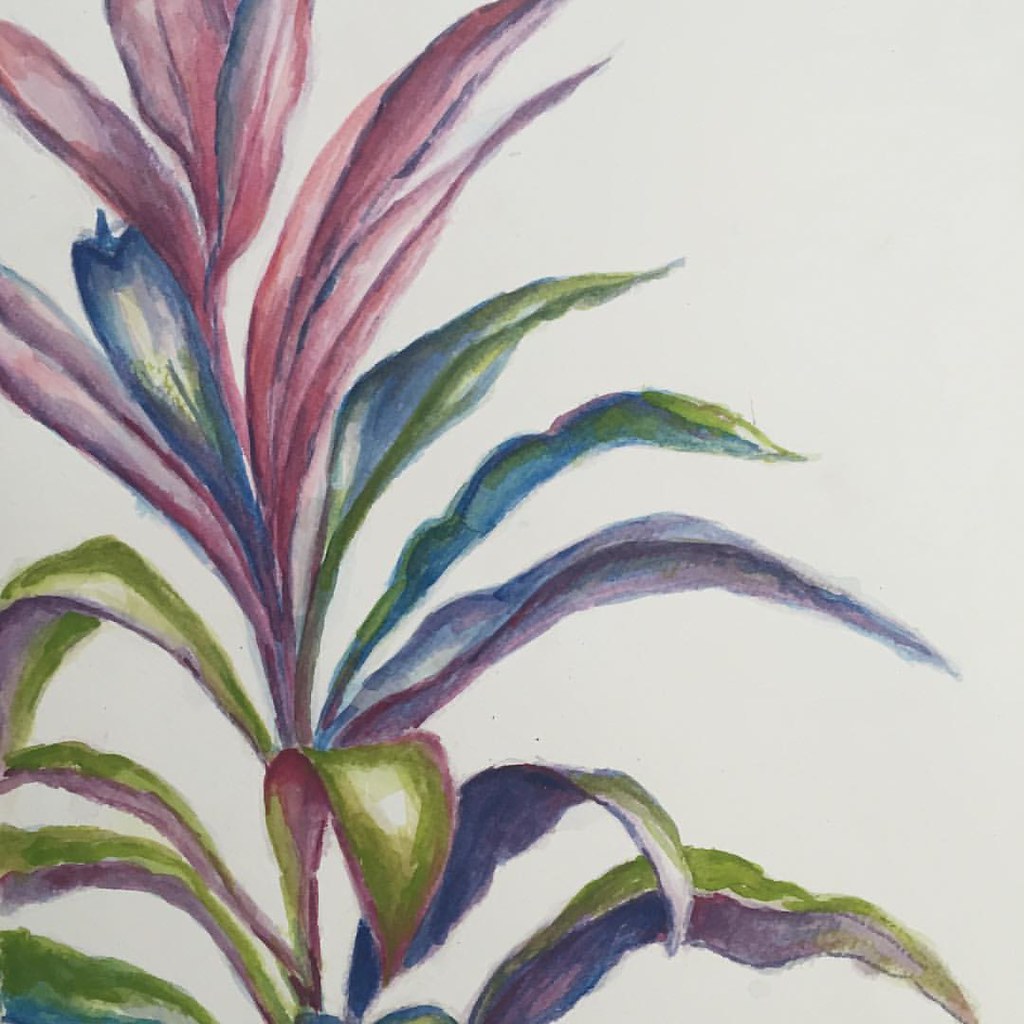This is an intricately detailed watercolor painting of a plant captured in a square, close-up photograph. The image is set against an off-white to dark cream background, emphasizing the vibrant colors of the plant. The plant itself starts at the bottom center-left where a pinkish-red stem rises vertically, splitting into long, thin, and pointy leaves that splay outwards. Each leaf showcases a gradient of hues—beginning with light greens and chartreuse on the lower left, transitioning to purples and blues in the middle, and culminating in striking pinks and blues at the top leaves. Some leaves are more richly colored with a variety of reds, yellows, and dark tones, exhibiting a realistic variegation reminiscent of a tea leaf plant. The leaves are depicted with both reflected white highlights and darker centers, creating a sense of depth. Throughout the painting, there is an elegant use of negative space that allows the intricate, pastel colors and wrinkled textures of the leaves to stand out brilliantly.